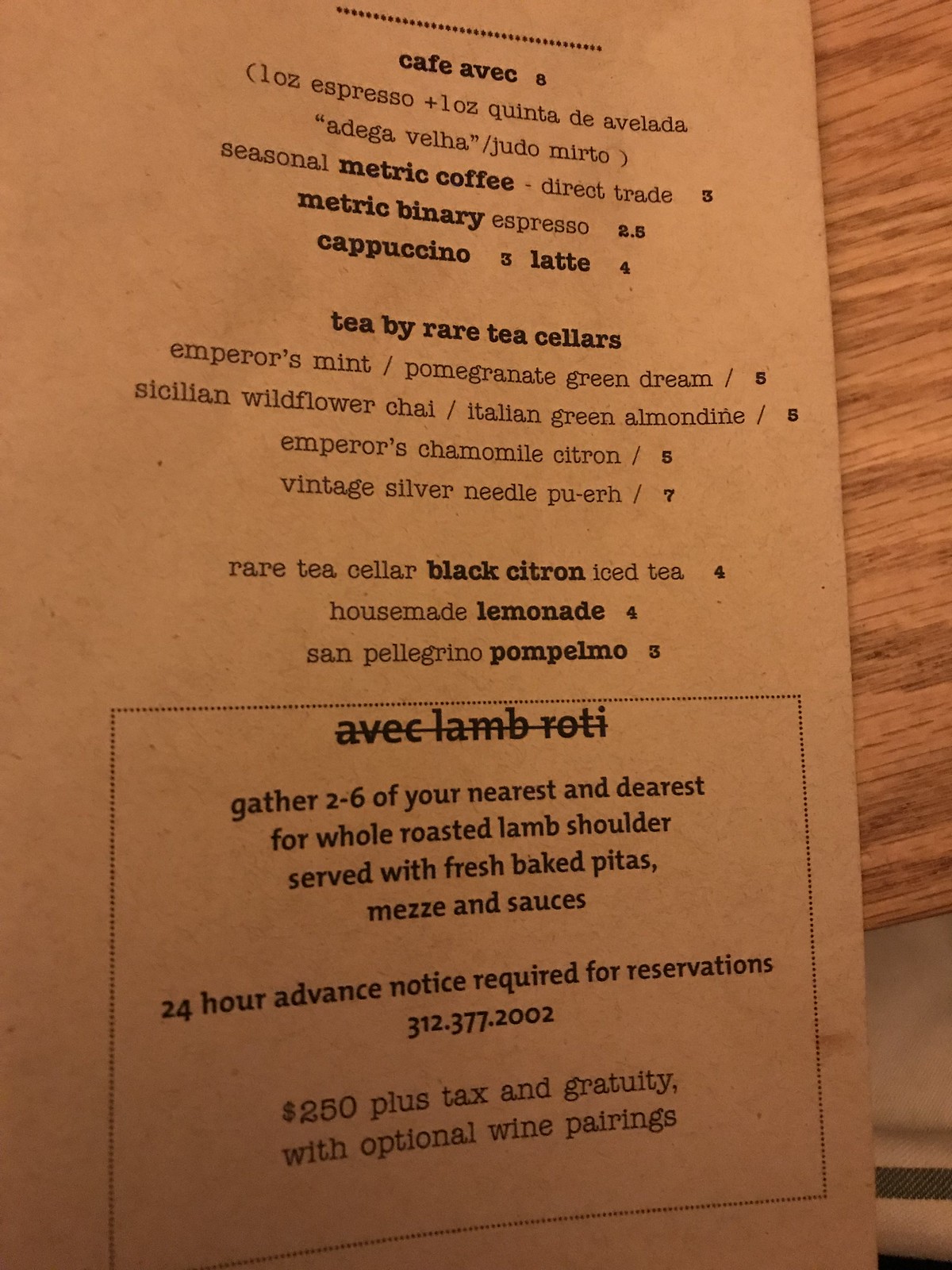The image depicts a light brown table with a slightly lighter-colored board situated below it. Resting on the table is a pale brown menu printed in black ink. At the top of the menu is a thin horizontal line followed by the title "Cafe Avek." Below the heading, the menu lists a detailed selection of beverages and teas:

- **Espresso and Coffee Selections**: One ounce espresso, one ounce Quinta de Avalada Adego, Veya, Udo, Mirto, seasonal Metric coffee, direct trade Metric Binary, espresso, cappuccino, and latte.
- **Teas by Rare Tea Sellers**: Emperor's Mint, Pomegranate Green Tea, Sicilian Wildflower Tea, Italian Green Almondine, Emperor's Chamomile Citron, Vintage Silver Needle Puring, and Rare Tea Seller Black Citron Iced Tea.
- **Other Beverages**: House-made lemonade and San Pellegrino Pompelmo.

At the bottom of the menu, there appears to be a description of a significant lamb dish. The clean, minimalist design of the menu emphasizes the quality and variety of the offerings at Cafe Avek.